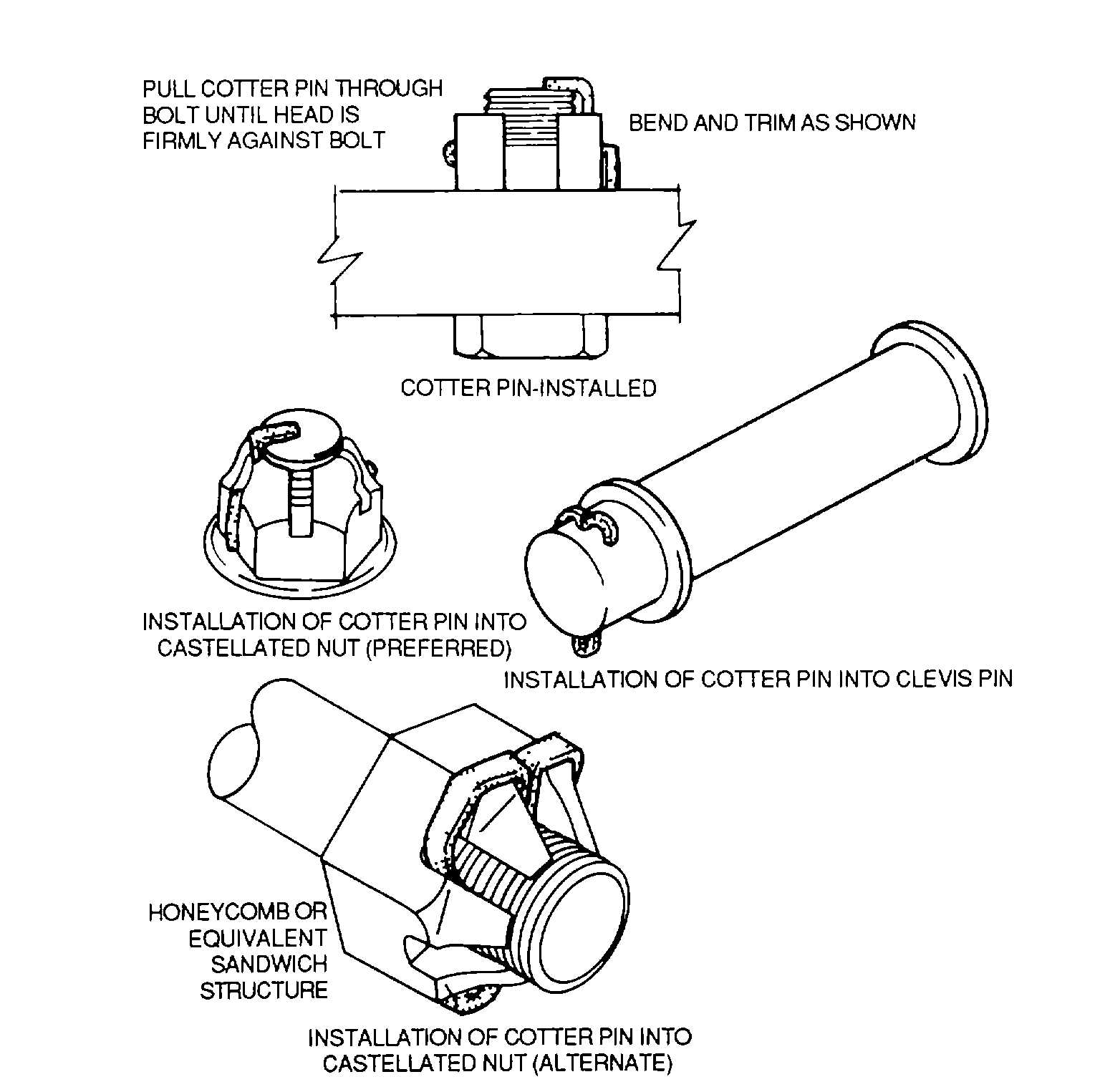This black-and-white diagram illustrates the installation process for cotter pins in various scenarios. The image comprises four distinct sections, each labeled with detailed instructions and descriptions. Starting from the top left, the diagram shows how to pull a cotter pin through a bolt until the head is firmly against the bolt, followed by bending and trimming the pin as indicated. The second part details installing a cotter pin into a castellated nut, which is marked as the preferred method. The third section explains the insertion of a cotter pin into a clevis pin within a honeycomb or equivalent sandwich structure. The final illustration, located on the lower left, describes an alternative method for installing the cotter pin into a castellated nut. Each section is accompanied by precise, step-by-step instructions that guide the user through the installation process, making the purpose of each component clear, even though the overall application may appear complex at first glance.